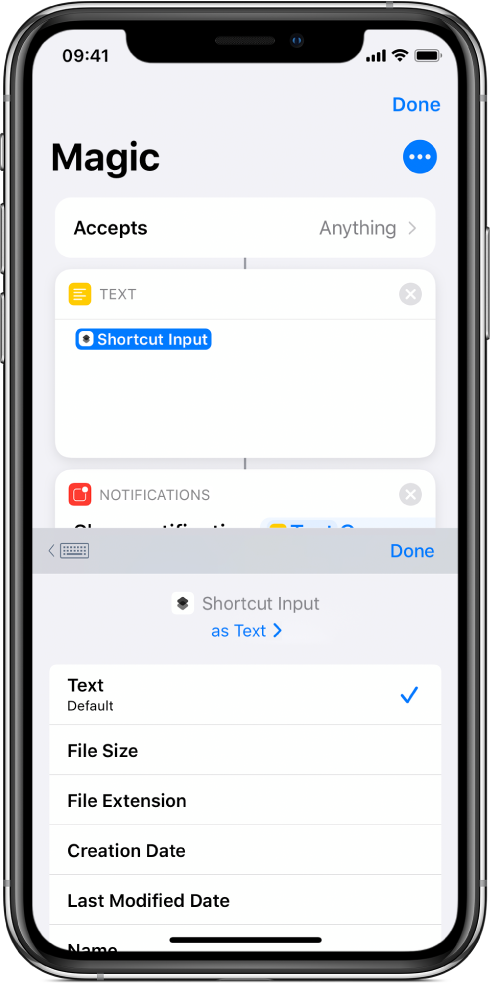A screenshot of a smartphone interface displaying a variety of interactive elements on a gray background. At the top, the time reads "9:41" with indicators for full battery life and strong Wi-Fi connection. Below the time, bold black text spells out "Magic." On the right side of this, there's a blue "Done" button and a blue circle containing three white dots aligned horizontally.

Further down the screen, there's an oval-shaped button labeled "Accept" in black text, currently grayed out with a right-facing arrow suggesting it leads to more information. Underneath this, a larger white rectangular box simply labeled "Text" sits adjacent to a yellow emoji made up of single white lines. 

Highlighted in blue, a "Shortcut Input" section is shown with a notification box partially visible below it. This notification box is red with an "X" for closing it, and nearby, a keyboard emoji is present.

Centered beneath this is another "Shortcut Input" text indicator in blue, featuring a right-facing arrow. At the bottom of the screen, there's a grouped list of selectable options, with "Text Default" checked in blue. Other options include file size, file extension, creation date, last modified date, and name, though some of these are cut off. The background is gray, while all dialog boxes and text boxes are white with black lettering.